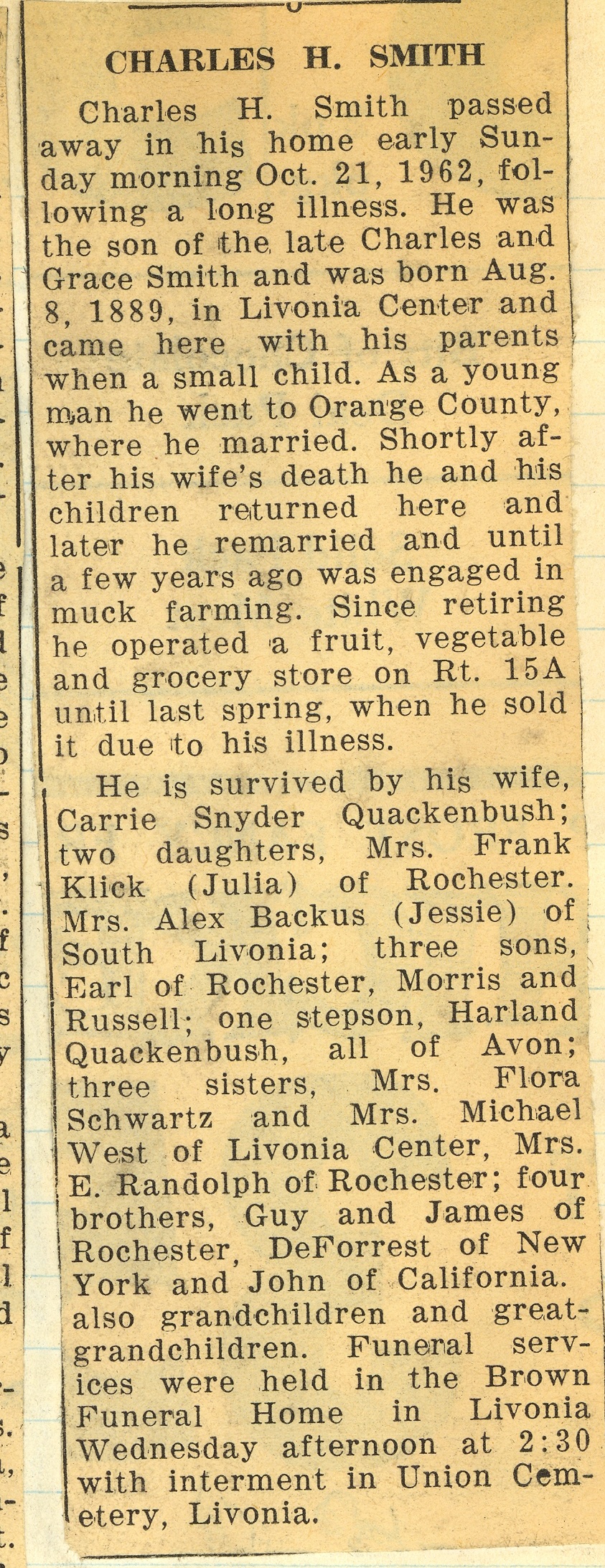This image showcases an aged, yellowed newspaper clipping of an obituary, laid atop a piece of notebook paper. The obituary, clearly cut out from an old, vintage newspaper, has black text across the top that prominently reads "Charles H. Smith" in bold letters. The obituary details that Charles H. Smith passed away in his home early Sunday morning, October 21st, 1962, following a long illness. Born on August 8th, 1889, in Livonia Center to the late Charles and Grace Smith, Charles moved to Orange County as a young man where he married. After his first wife's death, he returned with his children and later remarried. He was engaged in muck farming until a few years before his retirement, after which he operated a fruit and vegetable grocery store on Route 15A, selling it only last spring due to his illness. Charles is survived by his wife, Carrie Snyder Quackenbush, two daughters, Mrs. Frankulek Julia of Rochester and Mrs. Alex Buckus-Jesse of South Livonia; three sons, Earl of Rochester, Morris, and Russell; one stepson, Harlan Quackenbush of Avon; three sisters, Mrs. Forrest Schwartz and Mrs. Michael West of Livonia Center, and Mrs. E. Randolph of Rochester; and four brothers, Guy and James of Rochester, DeForest of New York, and John of California. Additionally, he is survived by numerous grandchildren and great-grandchildren. Funeral services were held at Brown Funeral Home in Livonia on Wednesday afternoon at 2:30, with interment following in Union Cemetery, Livonia. To the left of the central obituary, a small portion of another newspaper cutout is just barely visible.